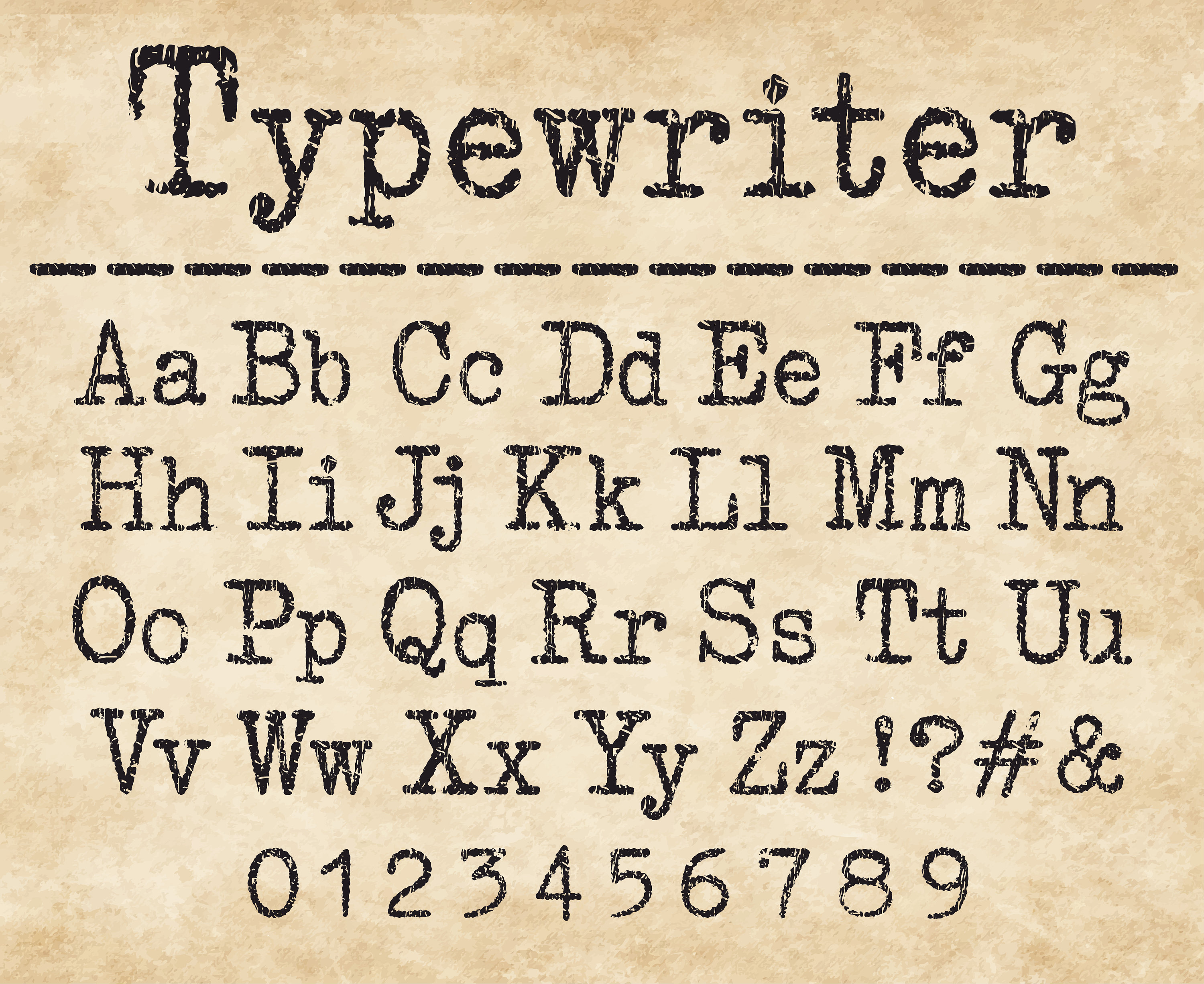This image depicts what appears to be a faded piece of paper with a beige or very light brown background. At the very top, the word "typewriter" is clearly printed in black ink. Directly below this, a dashed border separates the title from subsequent text. The main portion of the image features the full uppercase and lowercase alphabet, arranged in pairs from A/a at the top to Z/z at the bottom. Following the letters, a series of punctuation marks is placed in a row, including an exclamation point, a question mark, a pound sign, and an ampersand. At the very bottom of the image, numbers 0 through 9 are displayed in black text, maintaining the typewritten font style seen throughout the image. The overall aesthetic is consistent with typewritten text, imparting a vintage feel to the document.